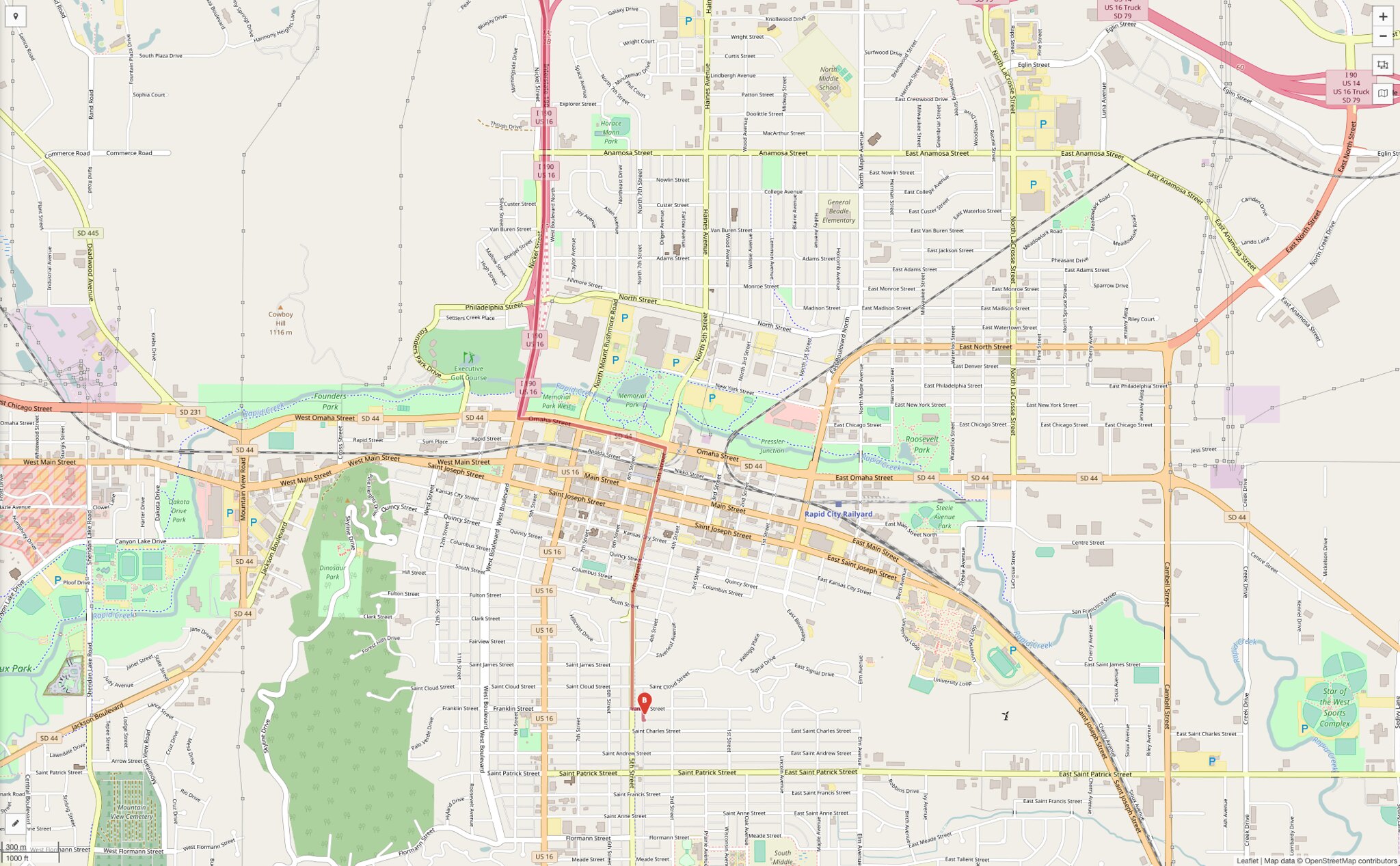A detailed map with various intricate elements occupies the frame, showcasing a blend of colors, lines, and symbols against a predominantly gray backdrop. In the upper left corner, a swath of gray is interspersed with light black lines, possibly indicating minor roads. To the left, a continuous yellow line suggests the presence of a significant highway traversing the map. A small purple box is situated at the bottom of this gray area, bordered by a green strip along the bottom.

A red line, potentially another major thoroughfare, slices through the map, delineating various sections. From the center to the far right, the map is awash with additional gray areas crisscrossed by black lines, likely representing a dense network of streets. At the lower part of this section lies an extensive green area paired with patches of yellow.

In the upper right corner, a thick red line diverges into three branches, close to a black symbol marked with a positive and negative sign, and flanked by two logos within white boxes. Nearby, a white line interconnects with the red one, splitting off to the left and right, navigated around by a yellow road. 

The bottom section from left to right is largely dominated by gray, with a prominent green stretch in the far left suggesting a forested area. Adjacent to this green expanse, additional green and red areas appear on the left. Scattered across the bottom middle, several thick yellow lines emerge, primarily branching towards the right, interspersed with more green areas, providing a dynamic and colorful overview of the map.